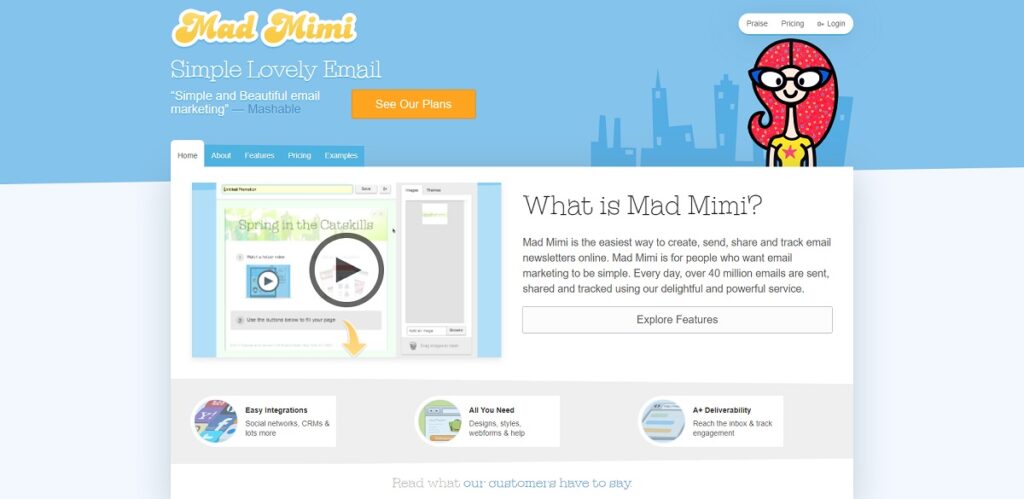"This image displays the desktop website of Madmeme, an email marketing service. The top section of the page features a navy blue background, which transitions into a lighter blue shade as you scroll down. Positioned at the top left corner is the Madmeme logo. Directly beneath the logo is the phrase 'Simply lovely email' in large, white letters. Below this phrase, a quote reads, 'Simple and beautiful email marketing' which is credited to Mashable. The Mashable credit is highlighted by a blue dash followed by 'Mashable' in blue font. To the right of the quote, there is a prominent orange button labeled 'See Our Plans.'

At the very top of the page, on the far right, there's a caricature of a woman with red sparkly hair. Above her caricature, a white navigation bar features links to 'Plans,' 'Pricing,' and 'Login.' 

In the center of the page, there is a mockup of the website displaying a play button at its center. To the right of the mockup, the text 'What is Madmeme?' is written in large gray letters, followed by a short informative paragraph explaining the service."